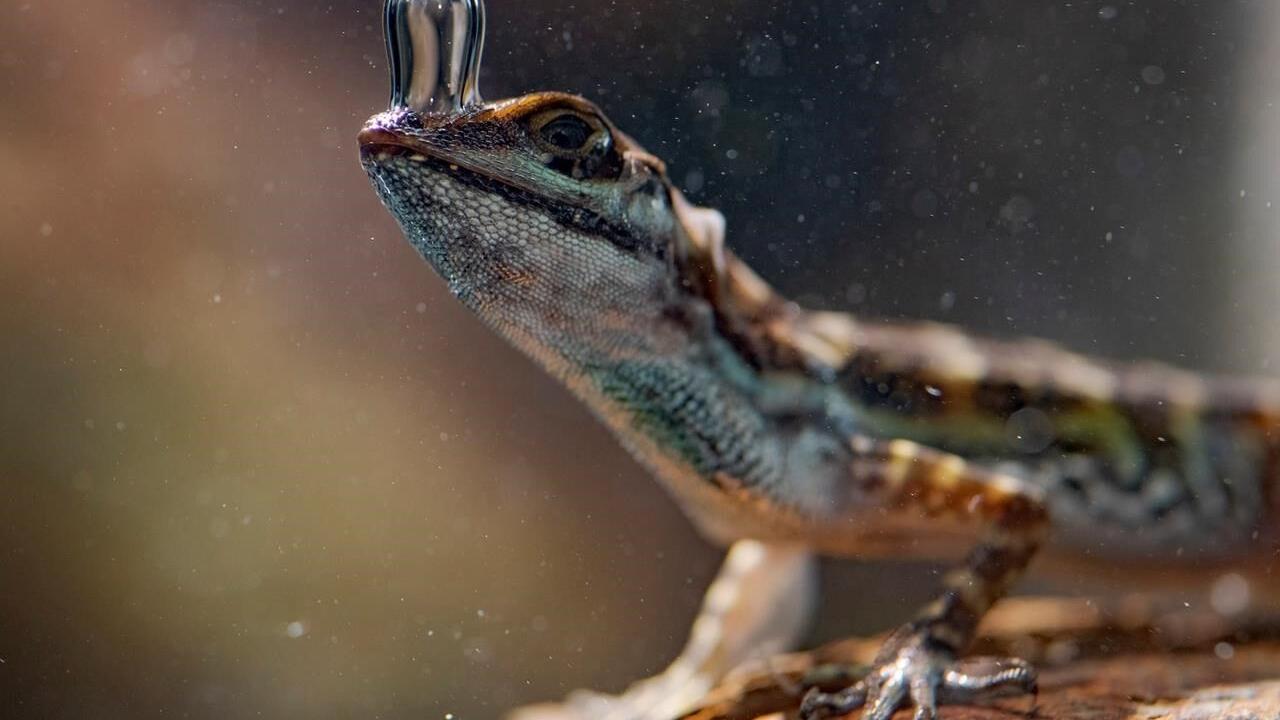This detailed close-up image showcases a lizard, possibly a gecko or an anole, characterized by a strikingly metallic, scaly body. The lizard's skin features an intricate mix of colors: copper hues on its head and back, yellow stripes along its body, a black line bordering its closed mouth, green scales on its chin, and a teal green underbelly. Its wide, alert black eyes gaze directly at the camera, emphasizing its vigilant posture.

A defining feature of the scene is a large, clear droplet of water precisely captured as it lands on the lizard's nose, flattening at the point of contact. The lizard's front legs, speckled with a combination of dark brown, yellow, green, and light gray, are clearly visible, emphasizing its scaly texture and sharp claws. The image also reveals blurred legs and body extending into the background, highlighting the creature's elongated form.

The background appears blurred, dotted with light spots and watermarks, suggesting the lizard is behind a glass surface, possibly in an aquarium. This glass has water stains, contributing to an impression of poor air quality, indicated by the extensive random particles floating around the lizard. The overall composition captures a moment of stillness and detail in the lizard's naturalistic habitat.